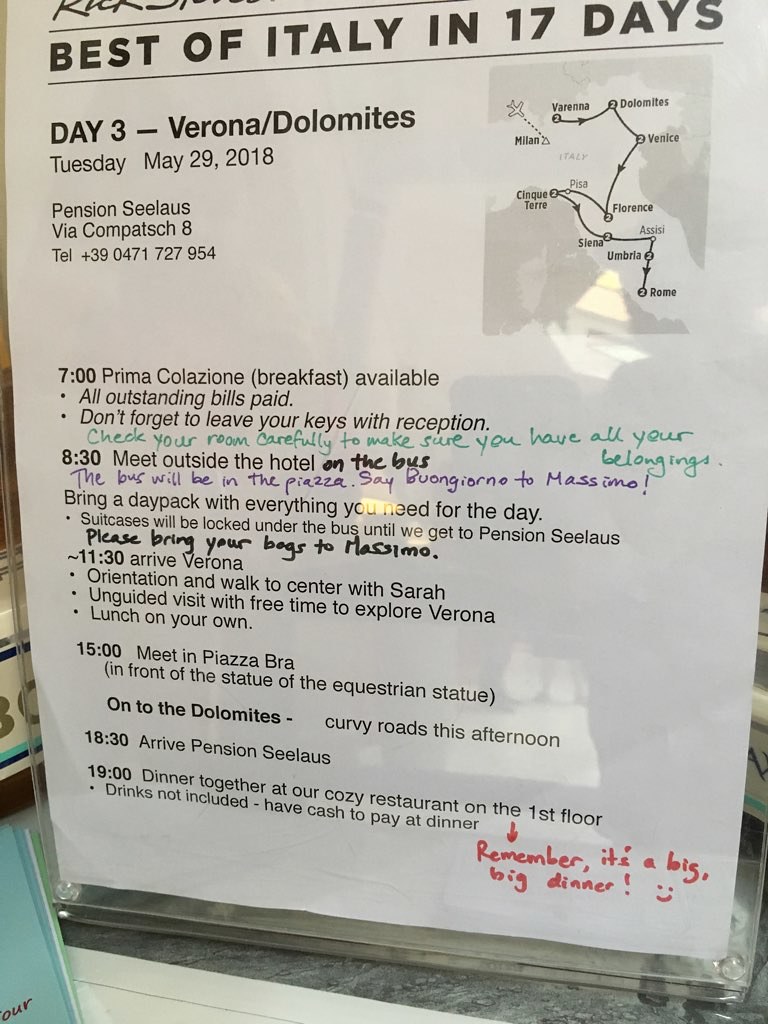The vertically aligned rectangular image depicts an itinerary for a 17-day tour titled "BEST OF ITALY IN 17 DAYS," displayed on a white piece of paper encased in a plastic stand, evident from reflections and the base at the bottom. The detailed schedule for "Day Three – Verona/Dolomites," dated Tuesday, May 29th, 2018, lists planned activities and logistics. The information starts with the accommodation details: "Pension Sileus, via Compatch 8, telephone 390471727954." 

Key scheduled events are:
- **07:00:** Primo Calzone breakfast available.
- **08:30:** Meet outside the hotel on the bus, which will be in the plaza; say "buongiorno" to Massimo. Guests should bring a day pack and hand their suitcases to Massimo, as they will be stored under the bus until the next stay.
- **11:30:** Arrival in Verona, followed by an orientation and walk to the center with Sarah. Free time for an unguided visit and lunch on your own.
- **15:00:** Meet in Piazza Bra, in front of the equestrian statue.
- **Subsequently:** Departure for the Dolomites via curvy roads.
- **18:30:** Arrival at Pension Sileus.
- **19:00:** Dinner together at the cozy restaurant on the first floor; drinks are not included, so have cash ready. A handwritten note in red at the bottom right corner emphasizes, "remember, it's a big, big dinner" with a smiley face.

On the upper right-hand corner of the paper, a small map outlines the travel route with an airplane icon indicating Milan, and connected dots marking stops in Venice, Florence, Siena, Umbria, and Rome. Further instructions mention checking out carefully and leaving room keys at reception.